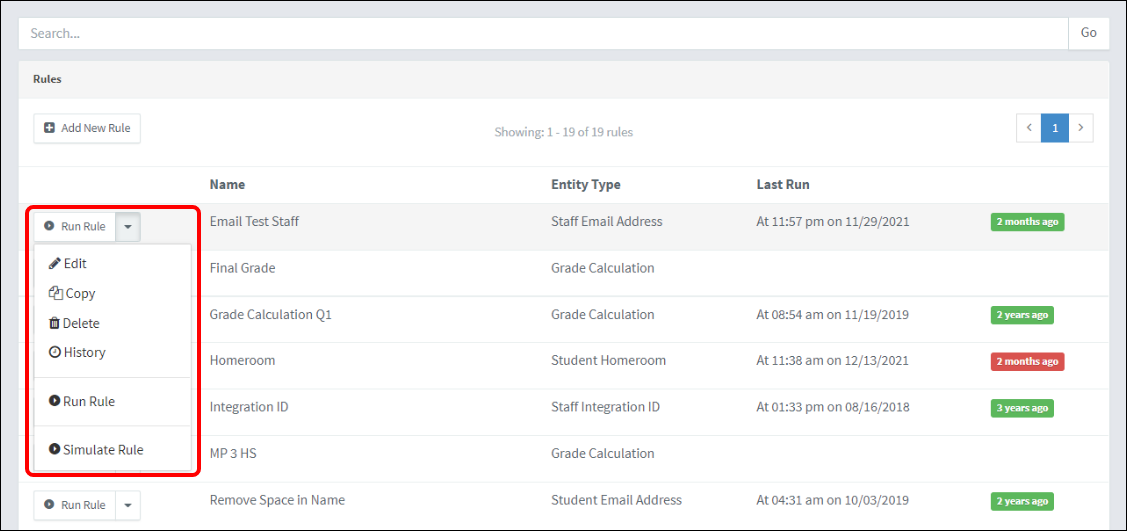The image is a horizontally rectangular screenshot of a user interface displaying a list of rules. The background is a narrow, light gray band surrounding the frame. At the top of the interface, there is a search field that extends the entire width of the frame, accompanied by a "Go" button on its right end.

Below the search field, on the upper left side, there is a heading labeled "Rules," under which a circular plus button is located, labeled "Add New Rule." Centrally positioned beneath these elements is a line of text stating "Showing 1 through 19 of 19 rules," indicating the total number of rules listed. To the right of this line, on the upper right side, the page navigation is displayed with the current page number "1" flanked by left and right arrow buttons for pagination.

Directly below these elements is a list with column headers categorized as "Name," "Entity Type," and "Last Run." To the left of the "Name" column, there's a section outlined in red, featuring a dropdown menu labeled "Run Rule." The dropdown menu options include "Edit," "Copy," "Delete," "History," "Run Rule," and "Simulate Rule," each accompanied by their respective icons.